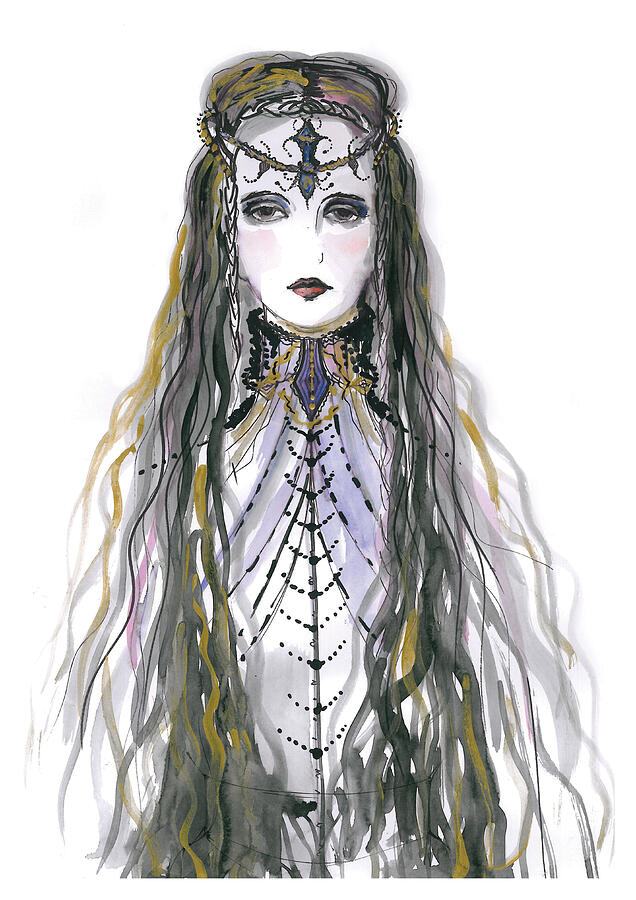This detailed illustration, resembling watercolor paint, portrays a goth woman with an ethereal, almost ghostly appearance. She is facing the viewer, her expression tired or bored, with droopy eyes accentuated by eyeshadow. Her lips are deep purple. Her skin is an extraordinarily pale shade, akin to antique white from Benjamin Moore, adding to her haunting allure.

Her long, straggly hair, a mix of gray and blonde, cascades down over her front, extending well below her waist and obscuring her arms and shoulders. Atop her head is a gold crown, adorned centrally with a scepter-like, diamond-shaped piece. 

She wears an intricate, spiderweb-patterned blouse that has a high choker collar, black near her neck, transitioning to a light lilac hue, then a more plain white as it moves down. The blouse features a design that descends into spiderweb-like buttons at the center. The image captures her just below the waist, allowing a clear view of the detailed and darkly elegant attire she adorns.